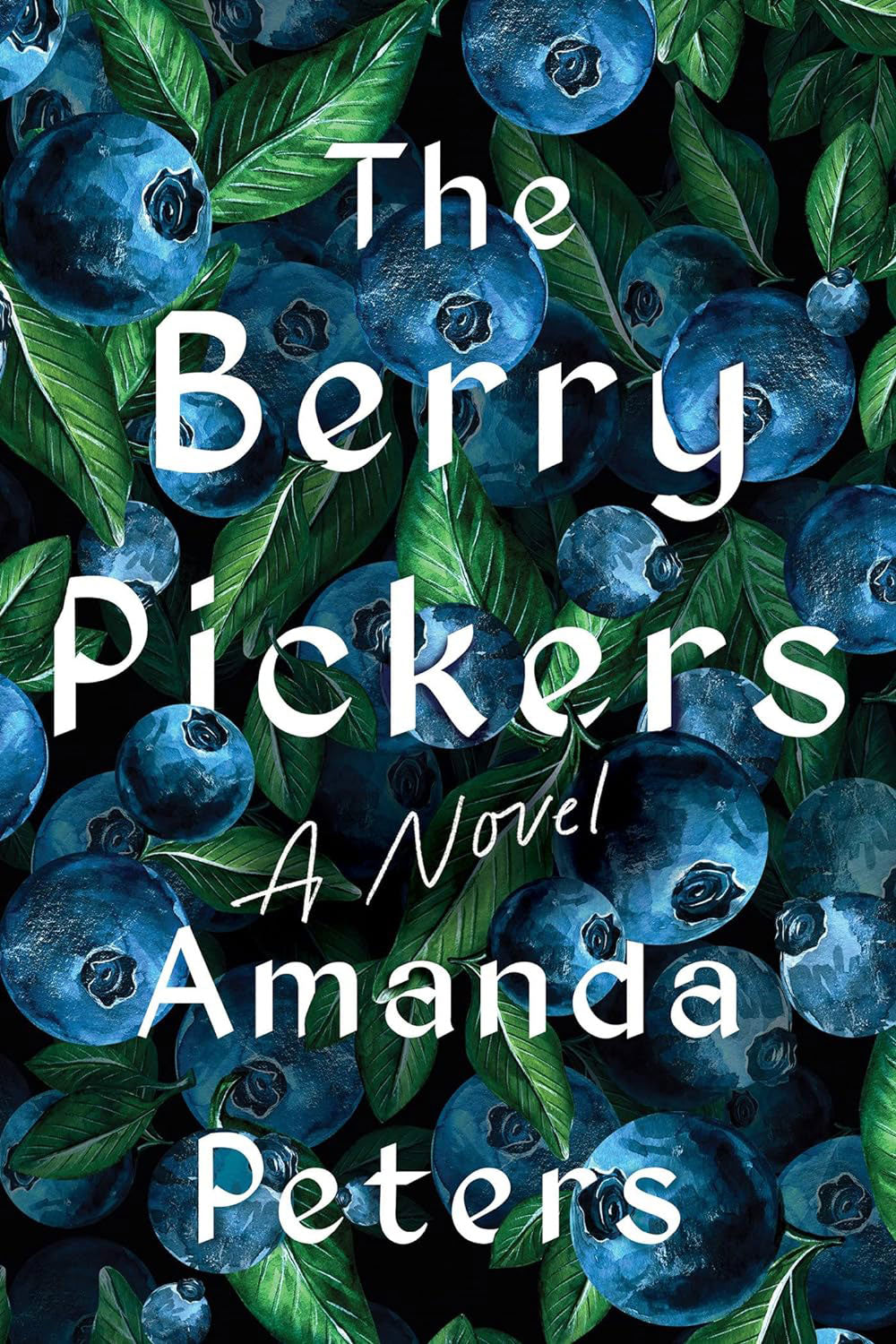The image showcases the front cover of a book entitled "The Berry Pickers," a novel by Amanda Peters. The title is written in white letters, with "The" at the top, followed by "Berry" and then "Pickers" in the middle of the cover. Below the title, in script, it reads "a novel," and at the bottom of the cover, the author's name, "Amanda Peters," is displayed. The background of the cover features a detailed and vibrant image of approximately 25-30 large, navy-colored blueberries hanging on the vine. The blueberries, with their characteristic shine and intricate details, including the little circles with jagged edges where they were picked, are interwoven with dark green leaves attached to the stems. The entire vertical, rectangular cover is filled with this lush, natural imagery, emphasizing the abundance and freshness of the berries.